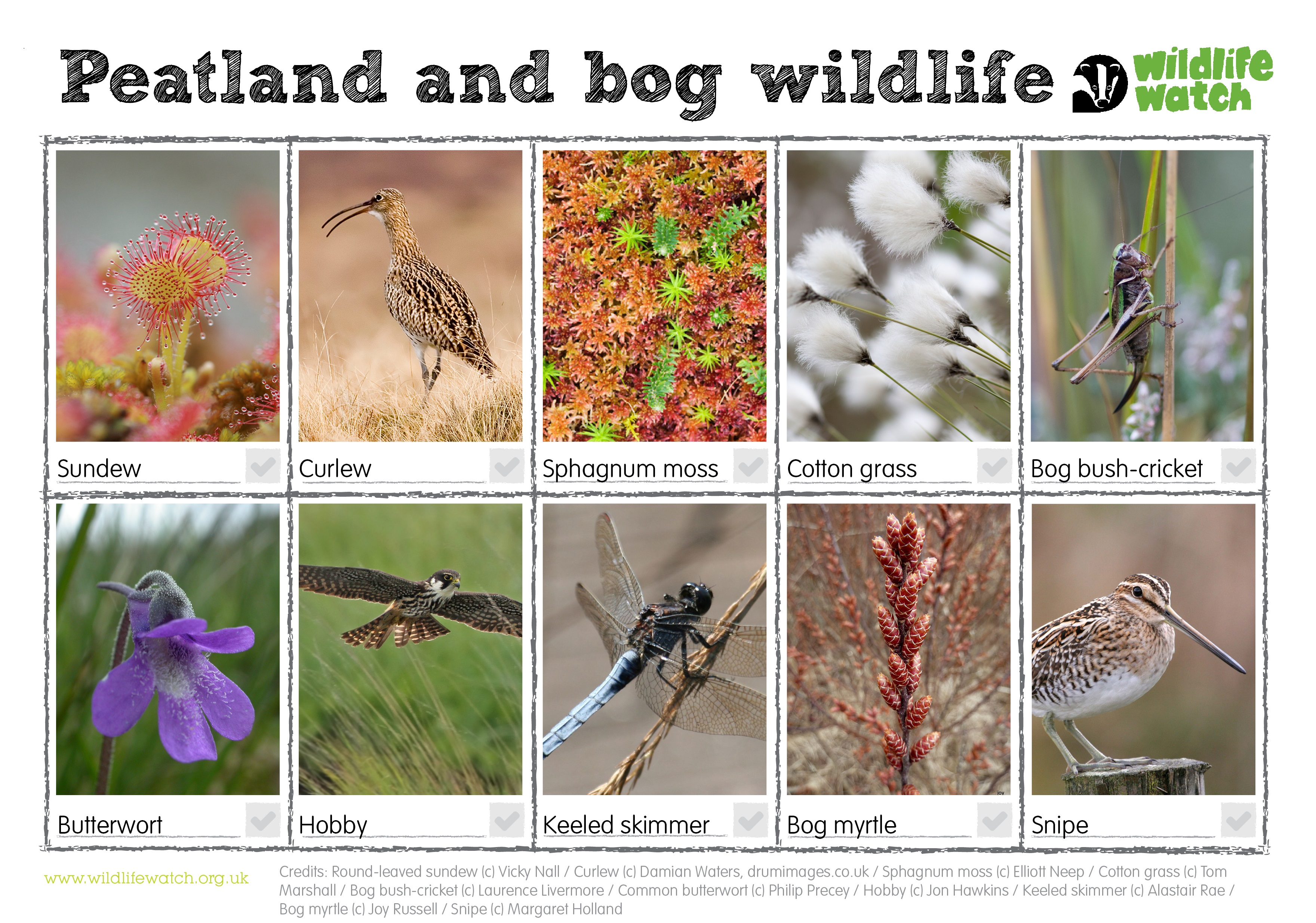The flyer titled "Peatland and Bog Wildlife" prominently features a logo with green lettering that reads "Wildlife Watch." It presents a detailed guide to various birds, plants, and insects in a ten-image collage. Arranged in two rows of five, each image is bordered in blackish-gray and includes a caption underneath. The top row showcases, from left to right, a sundew plant, a curlew bird, sphagnum moss, cotton grass, and a bog bush cricket. The bottom row depicts a butterwort flower, a hobby bird in flight, a keeled skimmer insect, bog myrtle, and a snipe bird. At the bottom of the flyer, the website "www.wildlifewatch.org.uk" is provided for further information.